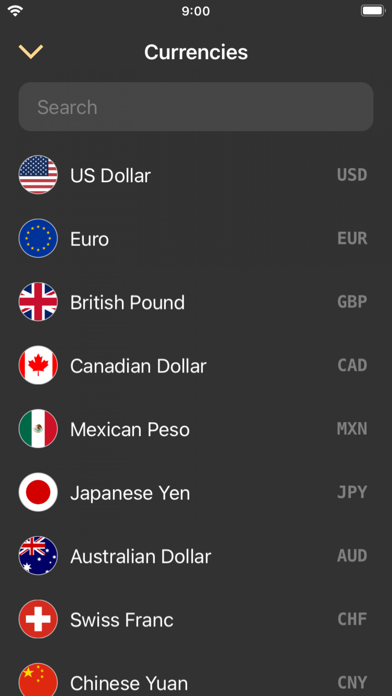The image depicts a screenshot taken from a cell phone. The background is entirely black. At the top of the screen, several indicators are visible: the current time displayed as "9:00", a fully charged battery icon shown in white on the right, and a Wi-Fi signal icon on the left. Below this are various currency exchange details divided into rows.

Each row on the left starts with a country's flag, followed by the name of its currency, and finally the currency code in gray font on the right. The first row features the United States flag, labeled "U.S. Dollar", with "USD" next to it. Below it, a blue circular flag represents the Euro, labeled "Euro" with "EUR" at the end. Following that is the United Kingdom's flag with a blue and white cross, labeled "British Pound" with "GBP" adjacent to it. Next is the Canadian flag with the red maple leaf, labeled "Canadian Dollar" with "CAD" on the right side. Each currency row follows this consistent pattern of flag, currency name, and currency code at the end.

A yellow downward-pointing arrow appears next to the U.S. Dollar row, likely indicating a selection or a drop in value.